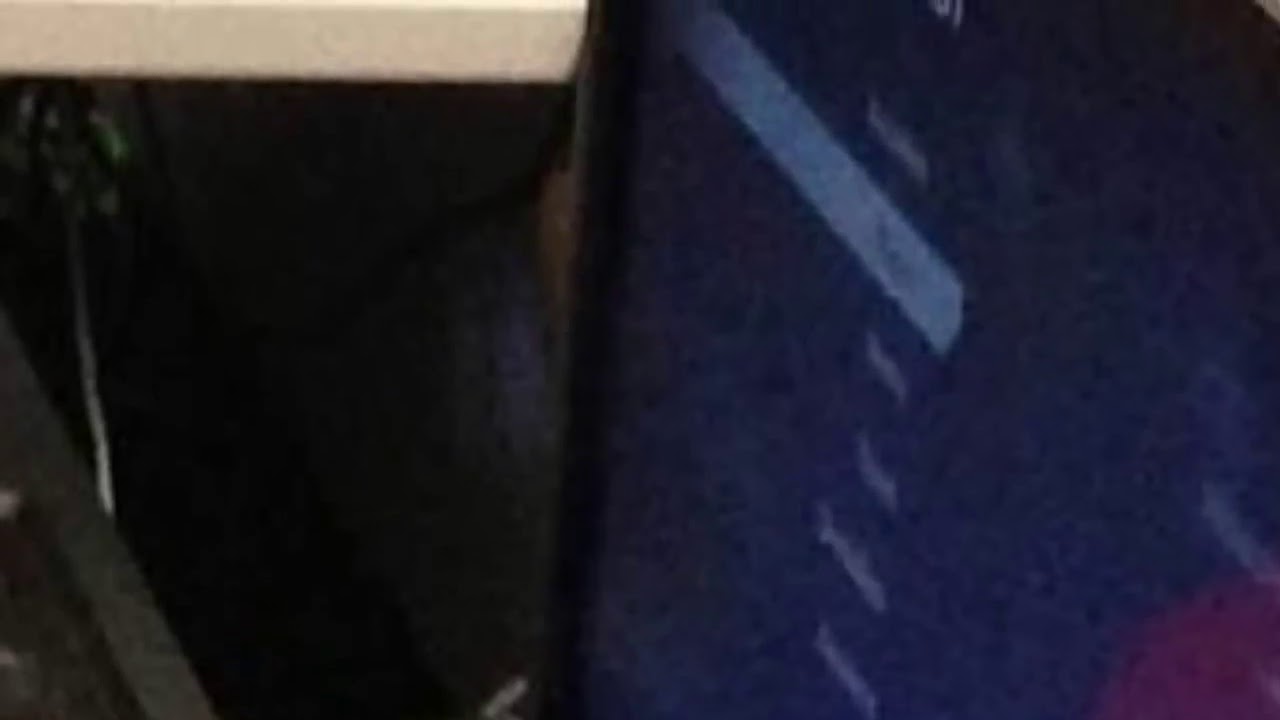The image is a grainy, close-up photo that is somewhat pixelated and blurry, making it difficult to identify its content clearly. The left side of the image features a vertical white stripe that could be part of an electronic device or appliance, possibly the side of a sink or the edge of a screen. Below this stripe, shadowy areas with dark gray and white lines suggest indeterminate structures. The right side, comprising roughly sixty percent of the image, displays a dark blue background with various thin white lines, reminiscent of a graphical user interface on a screen. One of these lines appears highlighted by a gray horizontal bar. In the lower right-hand corner, there is a faint, possibly reflective, purple quarter-circle shape. The blurred and poorly lit nature of the photo challenges the viewer to decipher its actual subject.